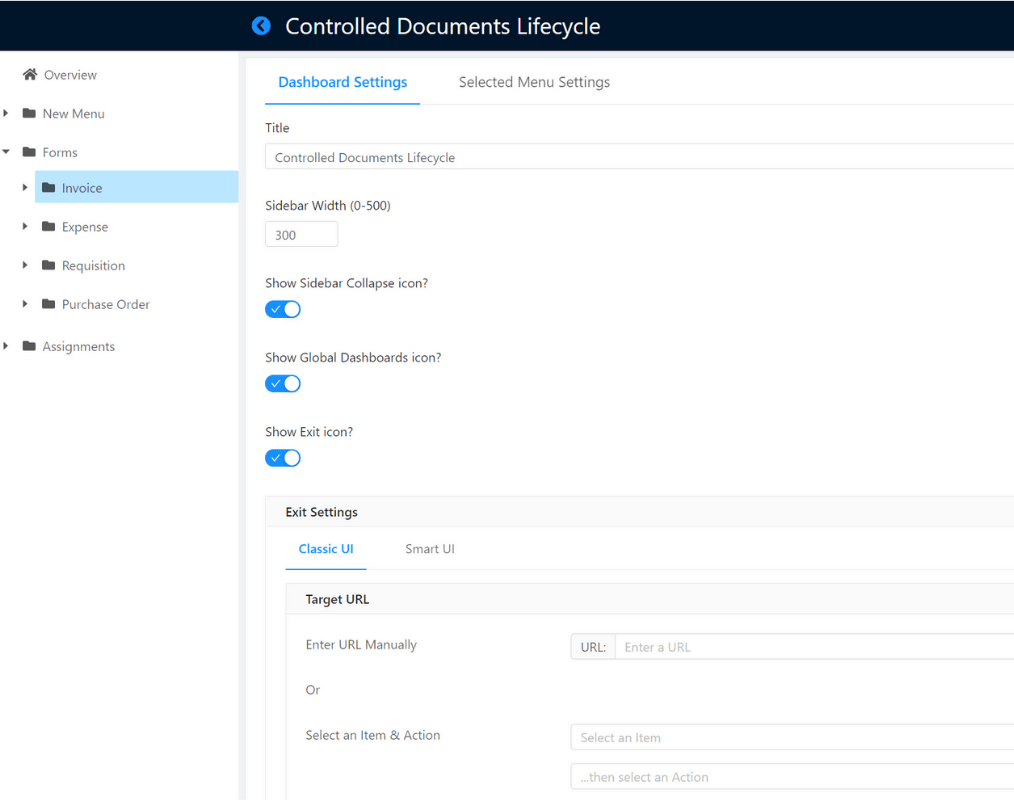The image depicts a detailed website interface with a dark, almost black banner at the top that veers slightly towards dark blue. Prominently featured on the banner is a round blue button with a leftward-pointing arrow, adjacent to the white text "Controlled Document Life Cycle."

Beneath the banner, a vertical menu is positioned on the left side of the page. The menu items include:
- Overview
- New Menu
- Forums
  - Invoice
  - Expense
  - Requisition
  - Purchase Order
- Assignments

To the right of the main menu, the page is labeled "Dashboard Settings" in blue text, followed by another label in gray text reading "Selected Menu Settings." Further down, additional settings are listed in blue text:
- Title: Controlled Documents Life Cycle
- Sidebar Width: 300
- Show Sidebar Icon
- Collapse Icon
- Show Global Dashboards Icon
- Show Exit Icon

Concluding the settings section are options for various UI and URL configurations:
- Exit Settings
- Classic UI
- Smart UI
- Target URL: Enter URL manually or select an item and action